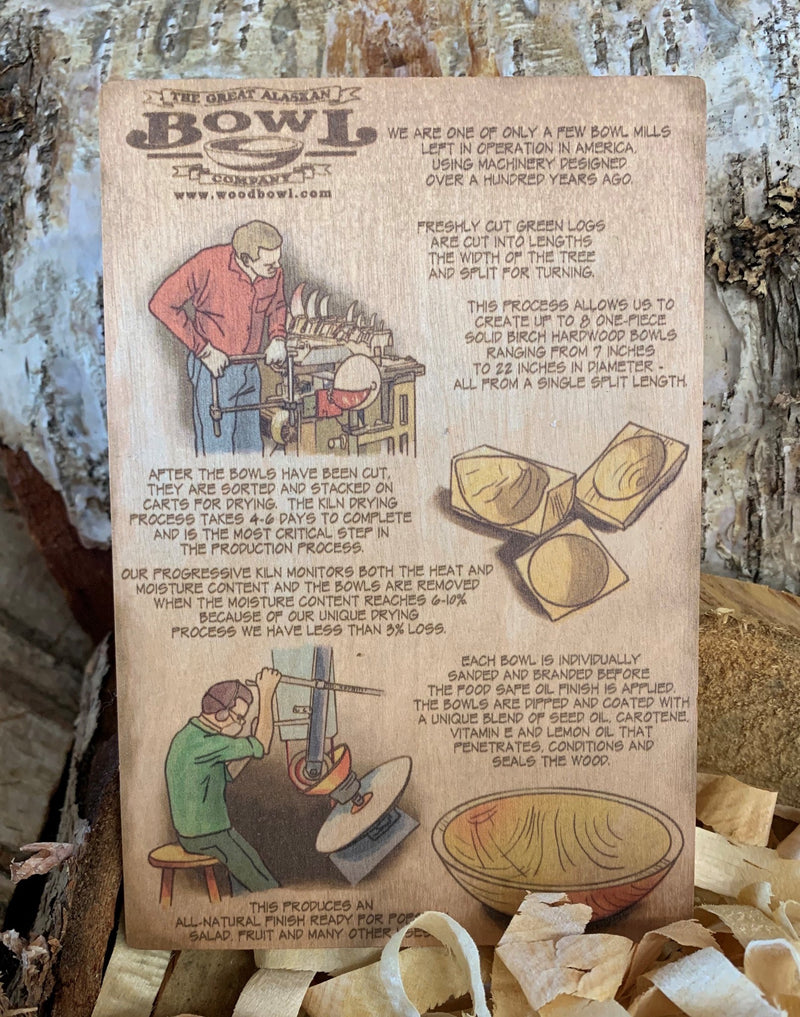The image showcases a beige, rectangular wooden board resembling a vintage poster or book cover. It prominently features “The Great Alaskan Bowl Company” in brown lettering alongside a dark brown illustration of a bowl. The overall background is a mix of light blue and dark cement texture.

The board includes several detailed illustrations depicting the bowl-making process. On the left, a man in a red shirt and blue jeans is shown operating machinery to carve bowls. Adjacent, there’s a step-by-step diagram illustrating bowl insert cutouts. Another illustration displays a man in a green shirt, wearing a face mask and protective ear coverings, engaged in sanding or grinding the bowls. Each scene underscores the craftsmanship and meticulous process involved in bowl creation.

Accompanying these images are paragraphs describing the traditional methods used by one of the few remaining bowl mills in America. The text emphasizes the use of century-old machinery and the process of turning freshly cut green logs into bowls.

At the very bottom, the board is nestled into a brown basket, surrounded by wood shavings, suggesting an ongoing woodworking activity. The board also includes a URL, www.woodbowl.com, indicating a modern touch to this otherwise classic presentation.